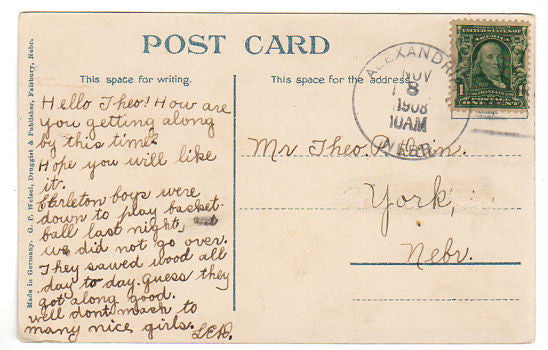This color image features an antique postcard from November 8th, 1908. The back of the postcard showcases a green one-cent stamp with Benjamin Franklin's portrait in the upper right corner. The postmark reads "Alexandria, November 8th, 1908, 10 AM" encircled around the date. The postcard is divided into two sections: on the left, there is blue vertical text stating "This space for writing," and on the right, "This space for address." The handwritten address is to Mr. Theo in York, Nebraska. The correspondent, signed as LED, writes in cursive: "Hello Theo, how are you getting along by this time? Hope you will like it. Charleston boys were down to play basketball last night. We did not go over. They sawed wood all day today, guess they got along good. Well, don't act too much to too many girls." The postcard bears a tactile sense of history, with its vintage handwriting and classic postal markings.